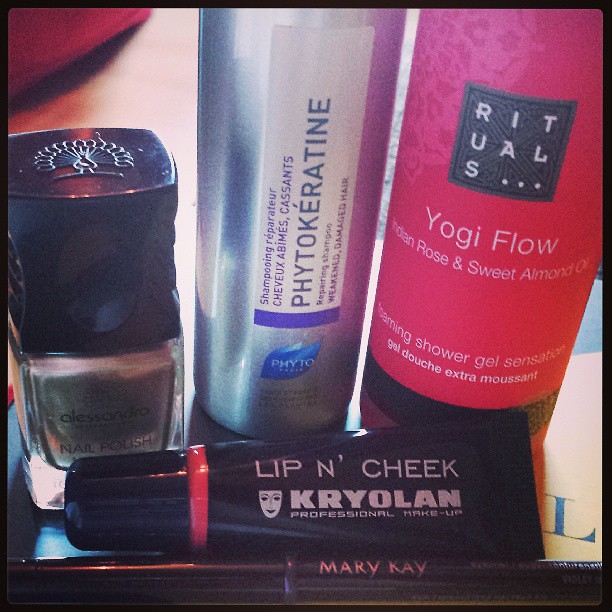This detailed photograph showcases a collection of five makeup and beauty products arranged on a table. 

Centered prominently is a red cylindrical bottle labeled "Rituals Yogi Flow" which features the fragrances of Indian rose and sweet almond oil. The black bottle with a wrap-around red label includes the words "shower gel sensation" in smaller text.

To the left of this bottle is a silver cylindrical bottle bearing the brand "Phyto." Its label emphasizes "Phyto Keratin" and highlights the product's function as a reparative shampoo for weakened, damaged hair, using a blue leaf symbol for identification.

Further to the left is a golden-hued nail polish bottle, distinguished by its black square lid topped with a peacock design. 

In the front row, a black tube of makeup labeled "Lip and Cheek" by Kryolan Professional Makeup is visible, sporting a thin line of pink near the lid and an icon resembling a face mask.

Adjacent to this tube lies a slender black pencil marked with "Mary Kay," completing the ensemble of beauty essentials showcased in this vibrant and detailed image.